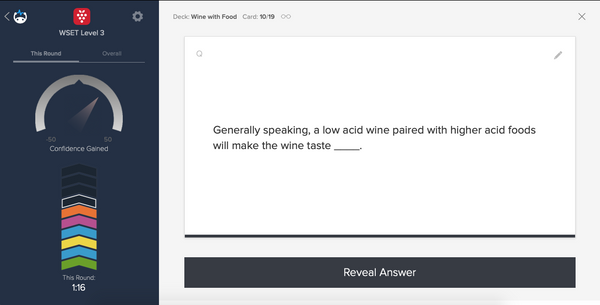On the left side of the image, there is a dark blackish-blue background with several elements layered on top. A gray arrow points to the right, followed by a white driving wheel. In the center, there is a wood-textured square with white dots resembling a strawberry pattern. Adjacent to this, there is a gray wheel.

Below these elements, there's text that reads "WSTE Level 3" followed by "This Round" and "Overall," indicating some metrics or levels. A graph arrow indicates "Confidence Gain," with markers at -50, 0, and +50, and a gray arrow pointing around the 25 mark. 

Beneath this, there are several solder patches: the first four are black, with the fourth encircled in white. The following patches are orange, pink, light blue, yellow, another light blue, and green. 

Further down, there is text in gray that states "This Round," with "1.16" written in white beside it. On the right-hand side, the text "Deck" in gray is accompanied by "Black, Wine with Food" in the same color. Below that, there is the word "Card" in gray, followed by a black "10-19." 

An infinity symbol appears in gray, and to the right, there's an X symbol. 

In the center of a white text box with a black border, black text reads: "Generally speaking, a low acid wine paired with higher acid foods will make wine taste" with a blank space for an answer. 

Below this, a red or blue line is visible, and within a blue square, white text reads: "Reveal Answer" prominently in the center.

This concludes the description. Moving on to the next image.